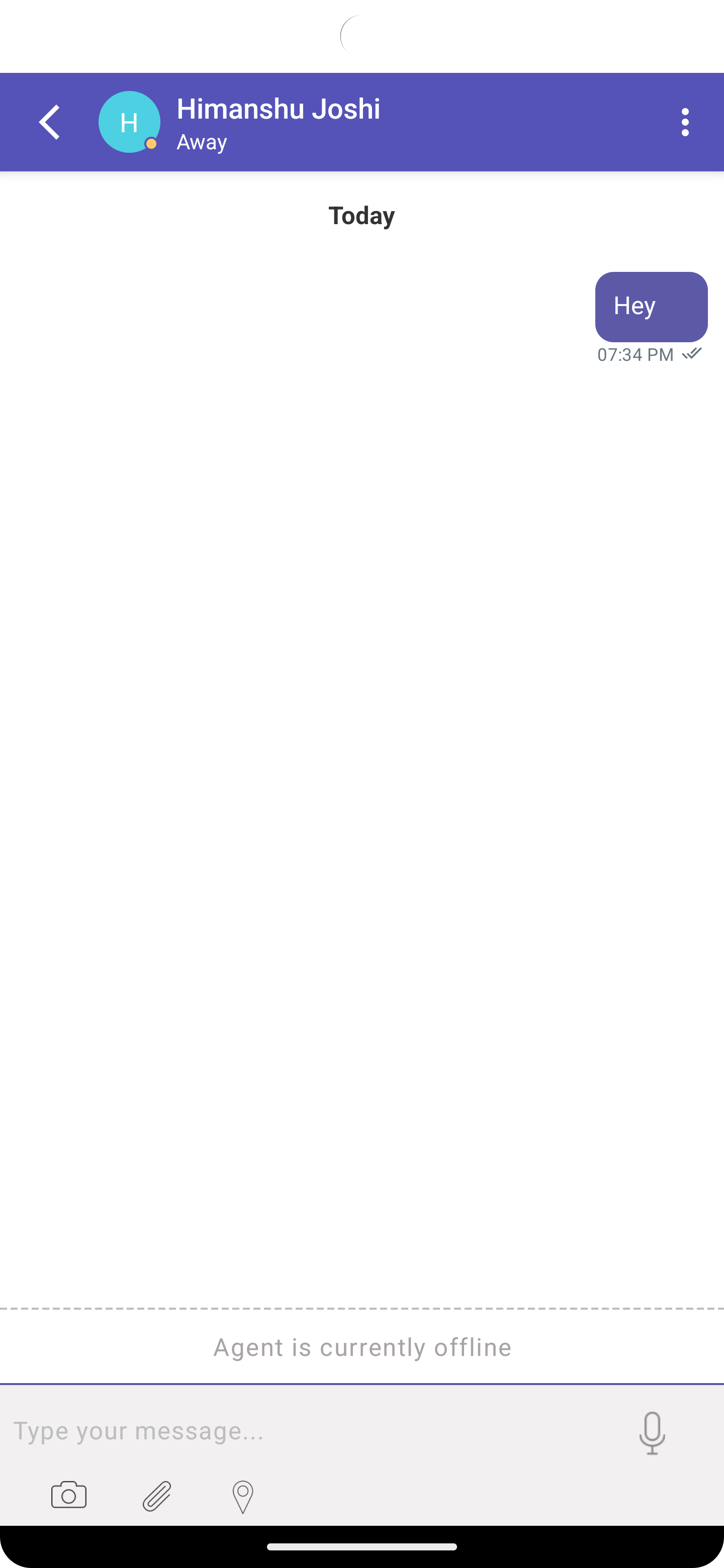This image is a mobile screenshot capturing a messaging app interface. The device has a tall, "candy bar" style screen with a faint line at the bottom, suggesting it's a newer Android or iOS phone. At the top, there's a black dot where the notification bar would usually appear, though the bar itself is hidden, likely concealed by the app.

The primary focus is a chat with a contact named "Himanshi Joshi," who is currently marked as "Away." The header features a back arrow on the left, a purple bar background behind the contact's name, and a trio of dots on the top right, presumably for additional options. 

The conversation so far includes a timestamp reading "Today, 7:34 p.m." followed by a double checkmark and the message "Hey," indicating the message has been seen. Below the message, there's a dotted line with the status "Agent is offline," then a solid horizontal line. Underneath, an input area displays a microphone icon with "Type your message," a camera icon, an attachment icon, and a location icon, indicating options to send voice messages, take or share photos, attach files, and share your location.

The rest of the chat history is blank, suggesting this message is either very recent or the conversation is just starting. The informality of "Hey" implies the sender might have a prior acquaintance with "Himanshi Joshi."

Overall, this screenshot seems to be from a professional or service-related app where users can interact with agents, who can be marked as online or offline and have functionalities for various media and location sharing.